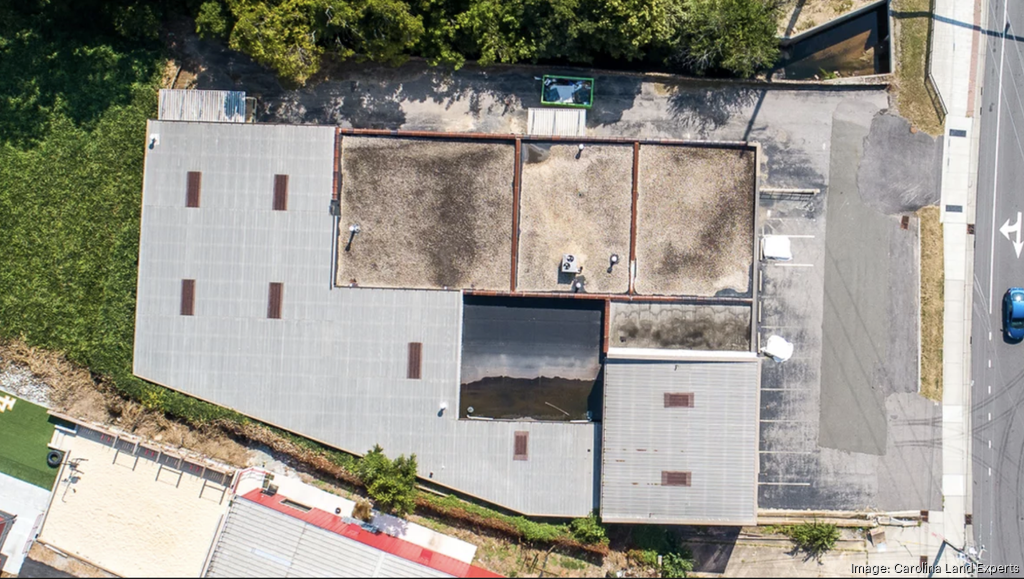The aerial overhead view, credited to Cardinalandexperts, shows a detailed scene of an industrial area during the day. Dominating the center of the image is a trapezoid-shaped building with a rooftop partially covered in gravel, featuring various sections divided by small walls and dotted with occasional AC units and small brown ventilation structures. The building is oriented facing right. A mostly empty parking lot extends from the right side of the building to the street on the extreme right, where a blue car is driving down. In front of the building, along the right side, are several small piles of white tarps or garbage occupying some parking spots. Beyond the building, to the top north side, a line of trees creates a natural barrier, while on the left side of the building, a grassy area stretches out. The bottom left corner of the image hints at an outdoor exercise area with a tire, bleachers, and the number four visible. Additional buildings can be seen adjacent to the main structure. The street runs from the top right to the bottom right of the image, completing the industrial and natural landscape depicted in the photograph.